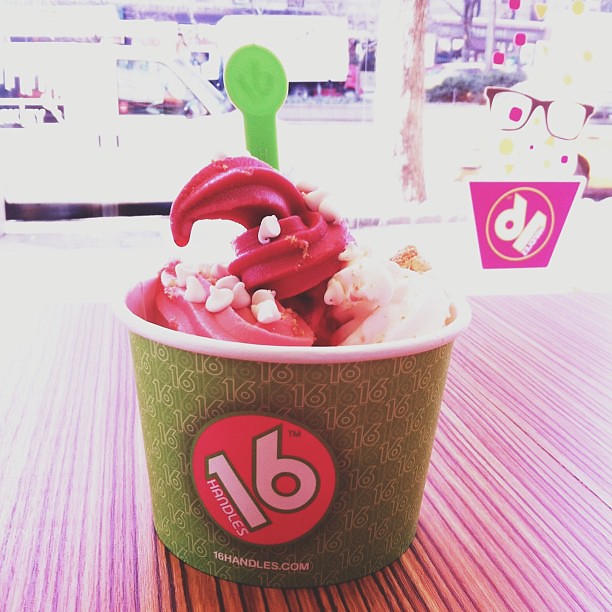This detailed photograph captures a close-up of a cup of soft serve ice cream, featuring a swirl of dark reddish-pink and white flavors, possibly fruit-based gelato. The ice cream is topped with white chocolate chips and other crunchy toppings partially visible in the background. The vibrant green paper cup bears the logo "16 Handles" in a red and white circle, with "16" prominently displayed. The background shows a blurred street scene with a white vehicle and faint glimpses of trees, suggesting the photo was taken from inside a shop. The table surface appears wooden, and there’s a hint of a sticker on the glass behind, with pink and purple stripes adding a colorful touch. Additionally, the website "16handles.com" is printed on the cup, emphasizing the branding. The image is brightly lit, possibly color-corrected for advertising purposes.